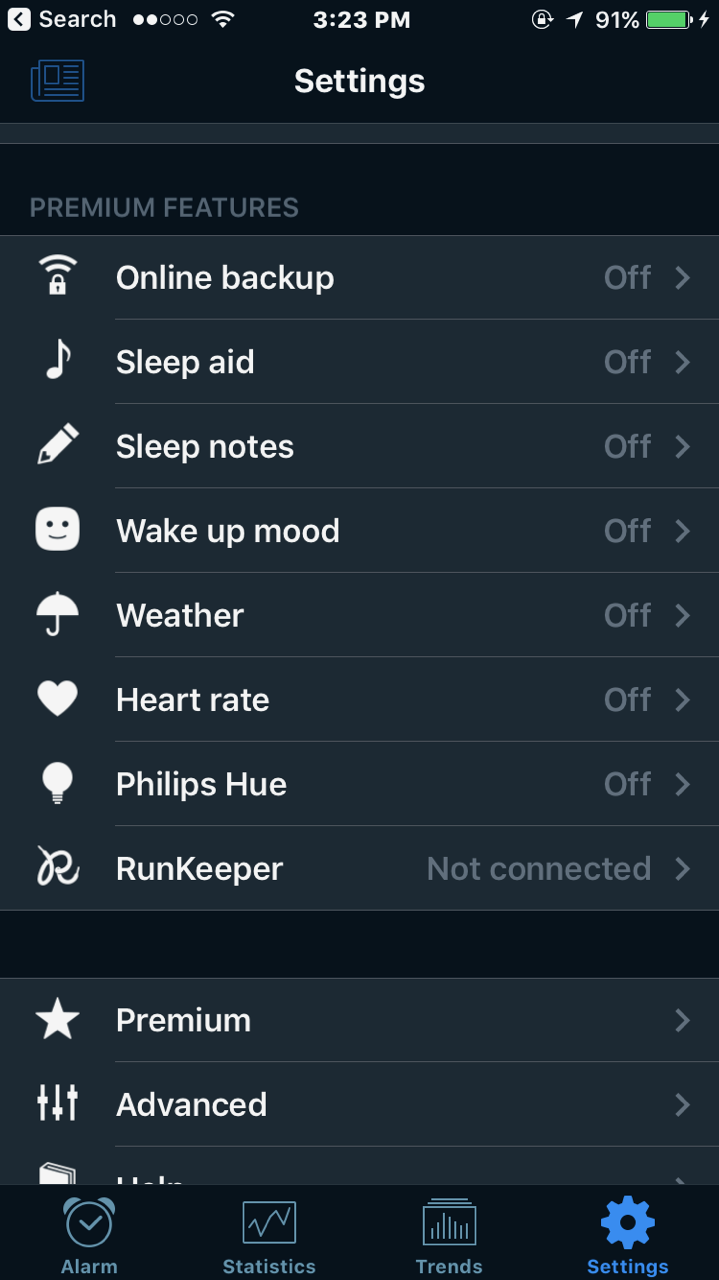The image displays a smartphone screen captured at 3:23 p.m. with 91% battery life remaining, either during a thunderstorm or while the battery is charging. The interface seems to be an application with premium features, characterized by a blue-themed newspaper style layout. The main display shows various functionalities and statuses including everything turned off, but highlights options for online backup, sleep aid, sleep notes, wake up mood, weather updates, heart rate monitoring, and connectivity to Phillips Hue and Runkeeper, which are currently not connected. The premium and advanced options are indicated with right arrows, however, some portions are cut off. The bottom of the screen features a black bar with blue clickable sections labeled "Alarm Statistics," "Trend Settings," and a darker blue option for "Settings."